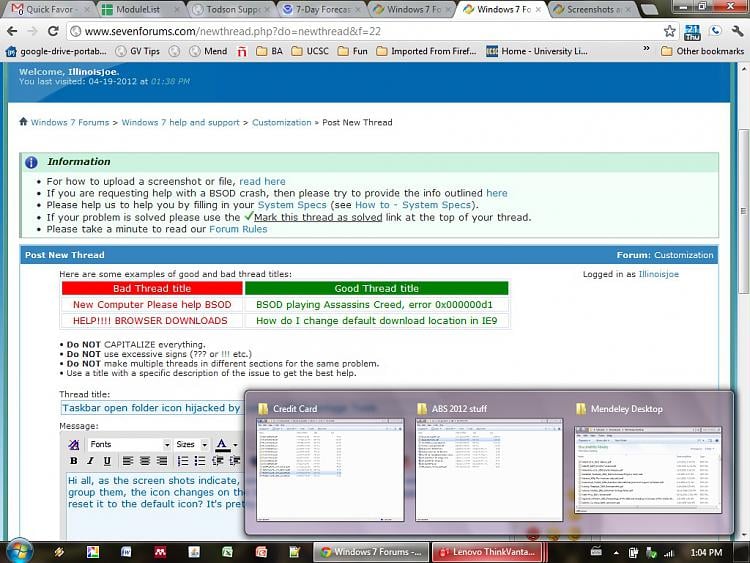The image depicts a detailed view of a computer screen, likely a laptop or desktop, displaying a browser with multiple open tabs. The uppermost portion of the screen reveals several tabs, with the first one on the left labeled "Quick Favor" possibly indicating an email. Adjacent to it, another tab is titled "Module Lists." Further to the right, a tab reads "TODSON" with the word "support" partially cut off. Additional open tabs include "7-Day Forecast," two separate tabs both for "Windows 7," one simply labeled "Screenshots."

On the right side of the screen, typical window control buttons – minimize, maximize, and close – are visible. The currently active tab, "Windows 7," displays the URL www.7forums.com. This website welcomes a user named Illinois Joe and provides information about their last visit. The page shown belongs to the "Windows 7 Forum," specifically under the "Windows 7 Help and Support" section.

The forum page provides instructions and examples for posting new threads, highlighting good and bad thread titles. Guidelines include avoiding full capitalization, excessive punctuation marks, and duplicates. There’s also a visible section labeled "Information" containing various informational snippets. At the bottom of the browser, the image captures parts of additional tabs related to "Credit Card," "ABS 2012 Stuff," and "Mendeley Desktop."

Overall, the picture gives an in-depth view of a user's multitasking setup in a browser with a focus on navigating and contributing to a tech support forum.